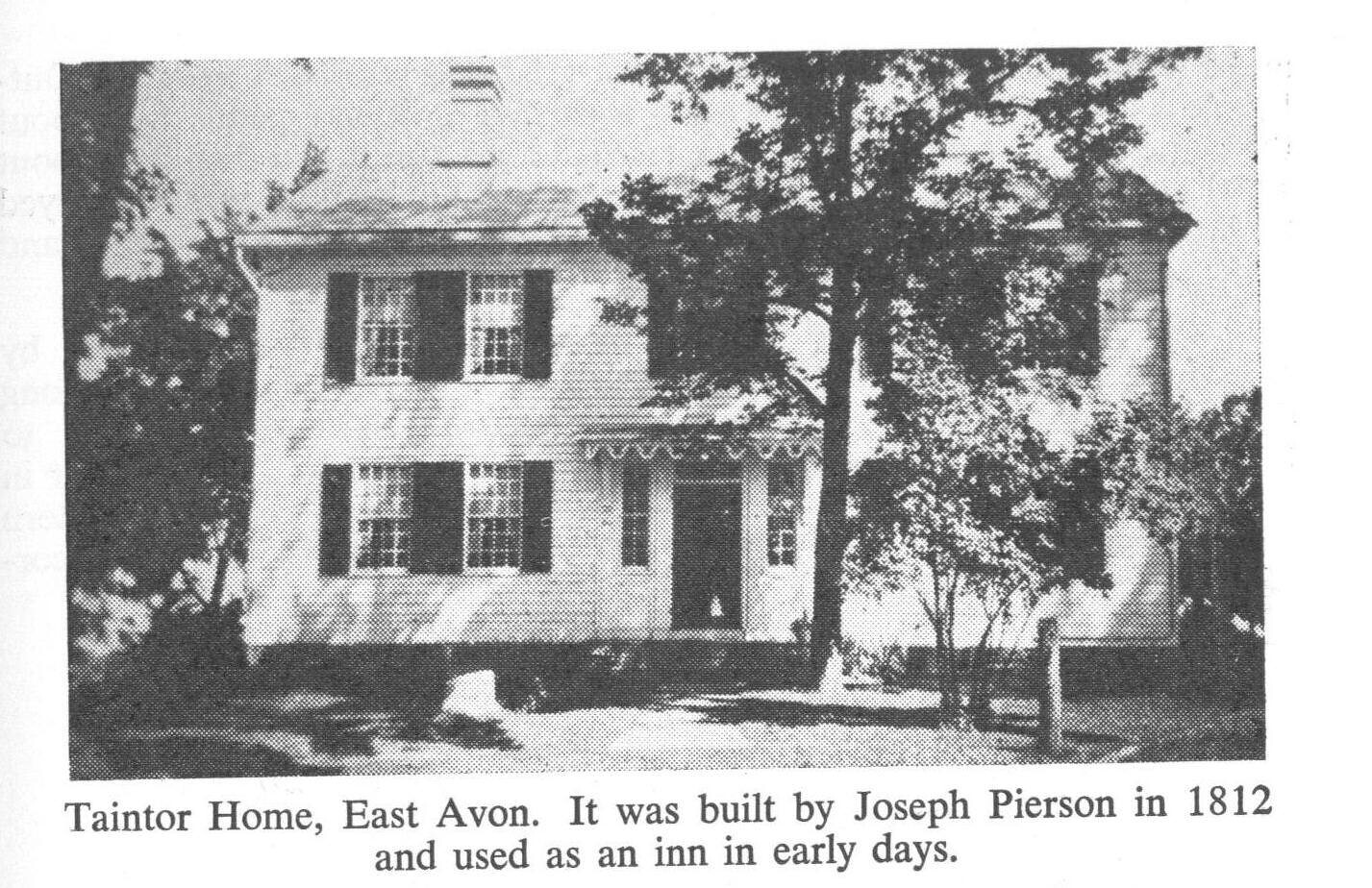This black and white photograph, resembling a newspaper clipping or a microfiche scan, depicts a historic two-story house identified as the Tainter Home in East Avon. Built by Joseph Pearson in 1812 and originally used as an inn, this residence features striking architectural details. The house boasts white siding, black storm shutters, and a dark front door with an awning. A chimney rises from the roof, which is bathed in sunlight, creating shadows from the surrounding trees. Among the trees in the front yard is a notably large one extending above the roofline, as well as a younger, thinner tree with leaves just starting to fill in, suggesting it may be springtime. The photograph is grainy, emphasizing its age and historical value, and it includes a caption in black text at the bottom: "Tainter Home, East Avon. It was built by Joseph Pearson in 1812 and used as an inn in early days." The classic, picturesque nature of the house is highlighted, hinting at its potential charm if seen in color. There may even be a hitching post in front of the house, adding to its historical authenticity.